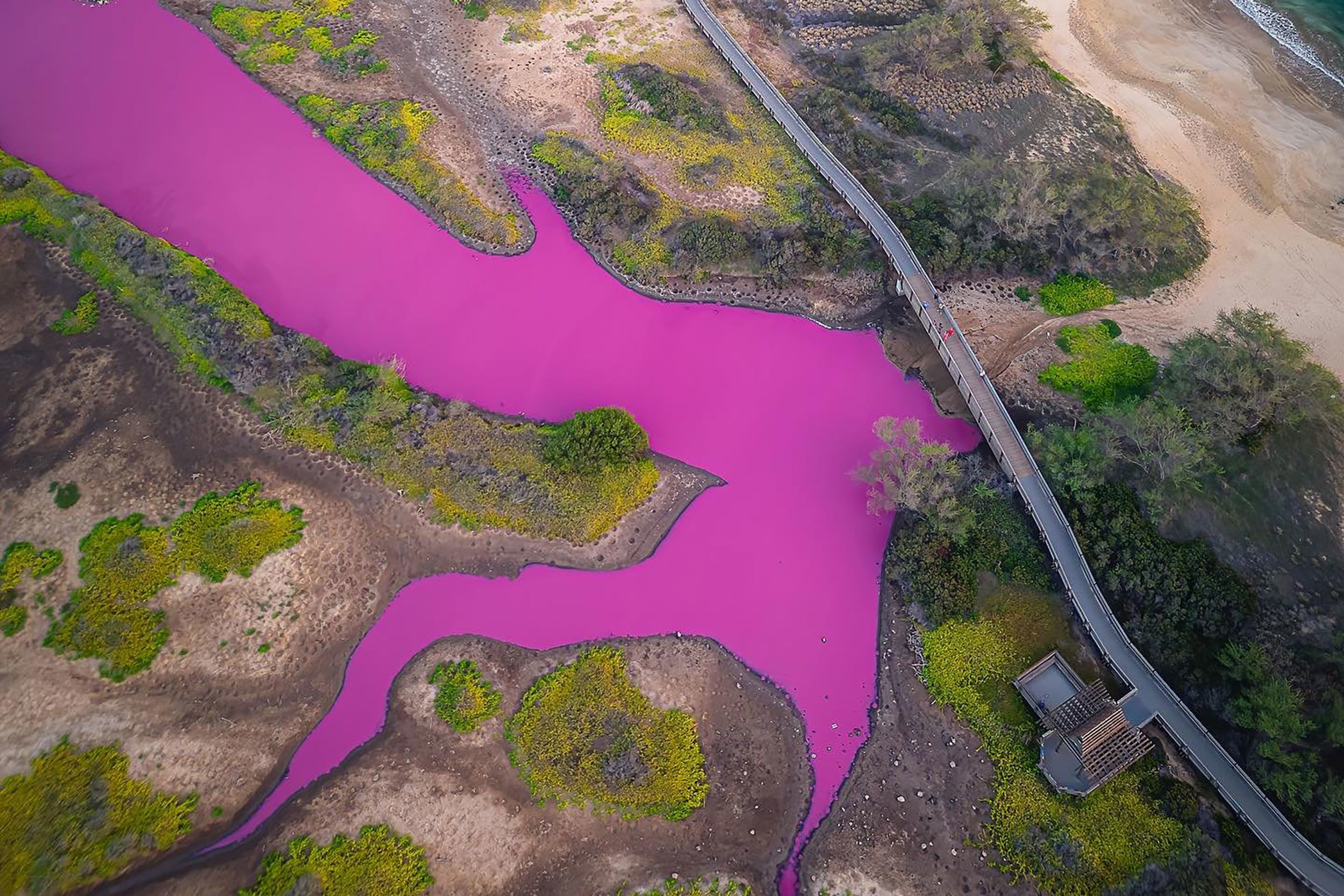This aerial photograph captures a striking landscape dominated by a vividly magenta or hot pink waterway winding through the terrain. With a direct downward angle, the image excludes the horizon, focusing instead on the peculiar features below. The body of water, colored naturally by algae, stands out as a stunning fuchsia or deep pink hue, resembling Pepto-Bismol. This pink river, possibly in Hawaii, contrasts sharply against the surrounding mixed landscape of sandy beaches, barren muddy patches, and bright green vegetation.

To the right of this striking pink waterway, a long bridge or walkway stretches across, populated by a few people, possibly bicycling or walking. Notably, the water stops just before it reaches under the bridge. Adjacent to the bridge, a small structure, perhaps a house or a station, is visible, adding to the sense of an inhabited but desolate area. Beyond this, a larger body of water—potentially an ocean or sea—appears in the upper right corner, suggested by the possible crest of a wave. The diverse ground textures and colors—ranging from earthy browns to vibrant greens—add to the visual complexity and allure of the scene.